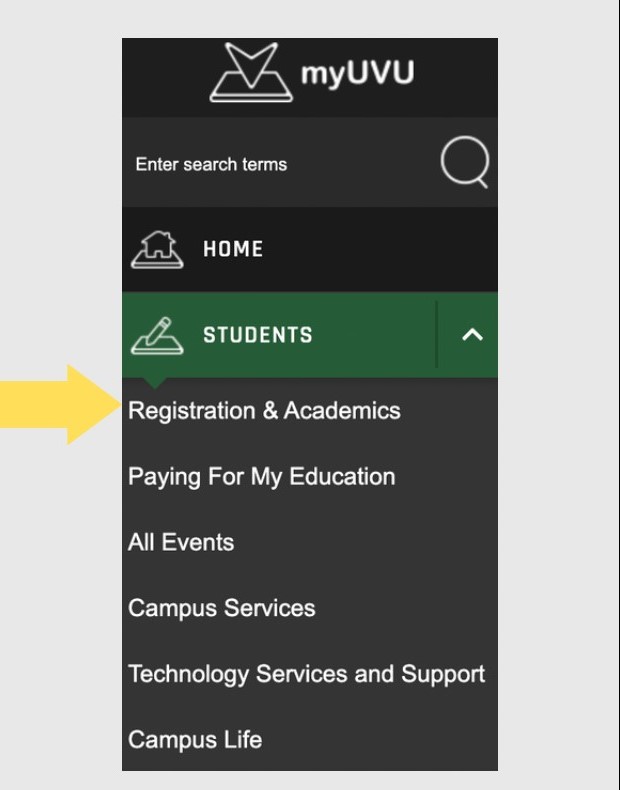The image features a detailed interface of the "My UVU" portal. The central visual element is a gray box enclosing a black box. At the top of this layout is an icon depicting a square, adjacent to which there is an arrow leaning on it, pointing towards the square. Beneath the arrow, the text "My UVU" is prominently displayed in all caps. Below this, there's a search bar with placeholder text reading "Enter search items." Accompanying this section is an icon of a question mark, and a home icon colored in black.

Highlighted within a green bar is a category designated for students, marked with upward-pointing arrows, indicating a possibly prioritized section. Adjacent to this is an icon of a piece of paper and a pen, presumably representing forms or documents. To the right of this green bar is a large yellow arrow that directs attention to "Registration." The sections following this, all in white text on a black background, include: "Academics," "Paying for My Education," "All Events," "Campus Services," "Technology Services and Support," and "Campus Life."

Despite the detailed categorization of various sections, there are no direct instructions or clickable links provided either at the top or the bottom of the interface, leaving ambiguity about the navigation process.